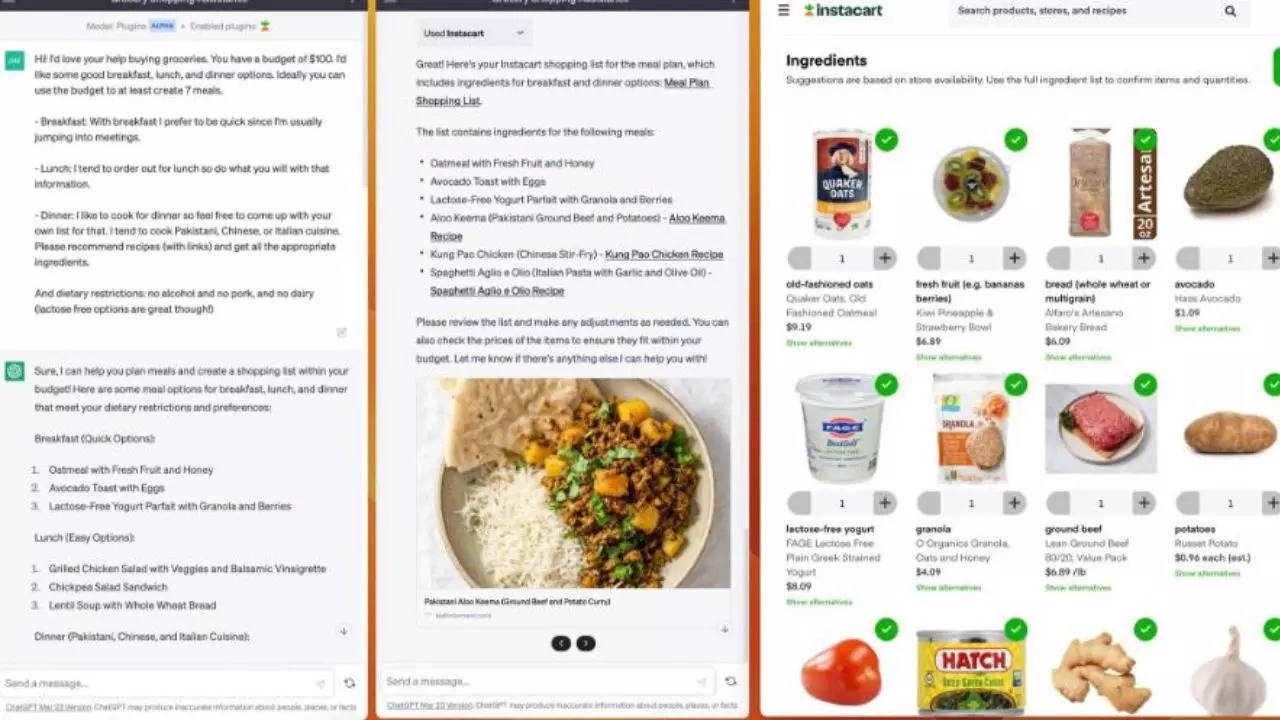**Detailed Caption:**

The image showcases a visually organized layout of three vertical screens, each long and thin, all related to foods and recipes. 

- **Left Screen**: This screen displays a text-based interaction where an individual has requested assistance with grocery shopping within a $100 budget. They express a need for seven meals covering breakfast, lunch, and dinner, with specific preferences and dietary restrictions: no alcohol, pork, or dairy, but lactose-free options are okay. Breakfast needs to be quick; lunch is typically ordered out; and for dinner, the individual enjoys cooking cuisines such as Pakistani, Chinese, or Italian. The response provides meal suggestions like oatmeal and avocado toast for breakfast, options like a grilled chicken salad and a lentil soup for lunch, and allows creative freedom for dinner.

- **Middle Screen**: This screen features a generated meal plan and shopping list. It further details the ingredients necessary for the suggested meals, such as oatmeal and avocado for breakfast, alongside recipes for dishes like Kung Pao chicken and spaghetti aglio e olio. The screen includes a visual of a balanced meal comprising meat, vegetables, and rice, illustrating one of the suggested dinner options.

- **Right Screen**: This screen presents an organized grocery list with corresponding images for each item. It includes various food items like Quaker oats, bananas, berries, bread, avocados, potatoes, ground beef, granola, lactose-free yogurt, and tomatoes, among others. Each item is shown with a clear, identifiable picture, likely part of an online shopping interface like Instacart, making it user-friendly and visually appealing.

The overarching theme of the three screens combined is a cohesive and detailed approach to meal planning and grocery shopping within a budget, tailored to specific dietary needs and preferences.